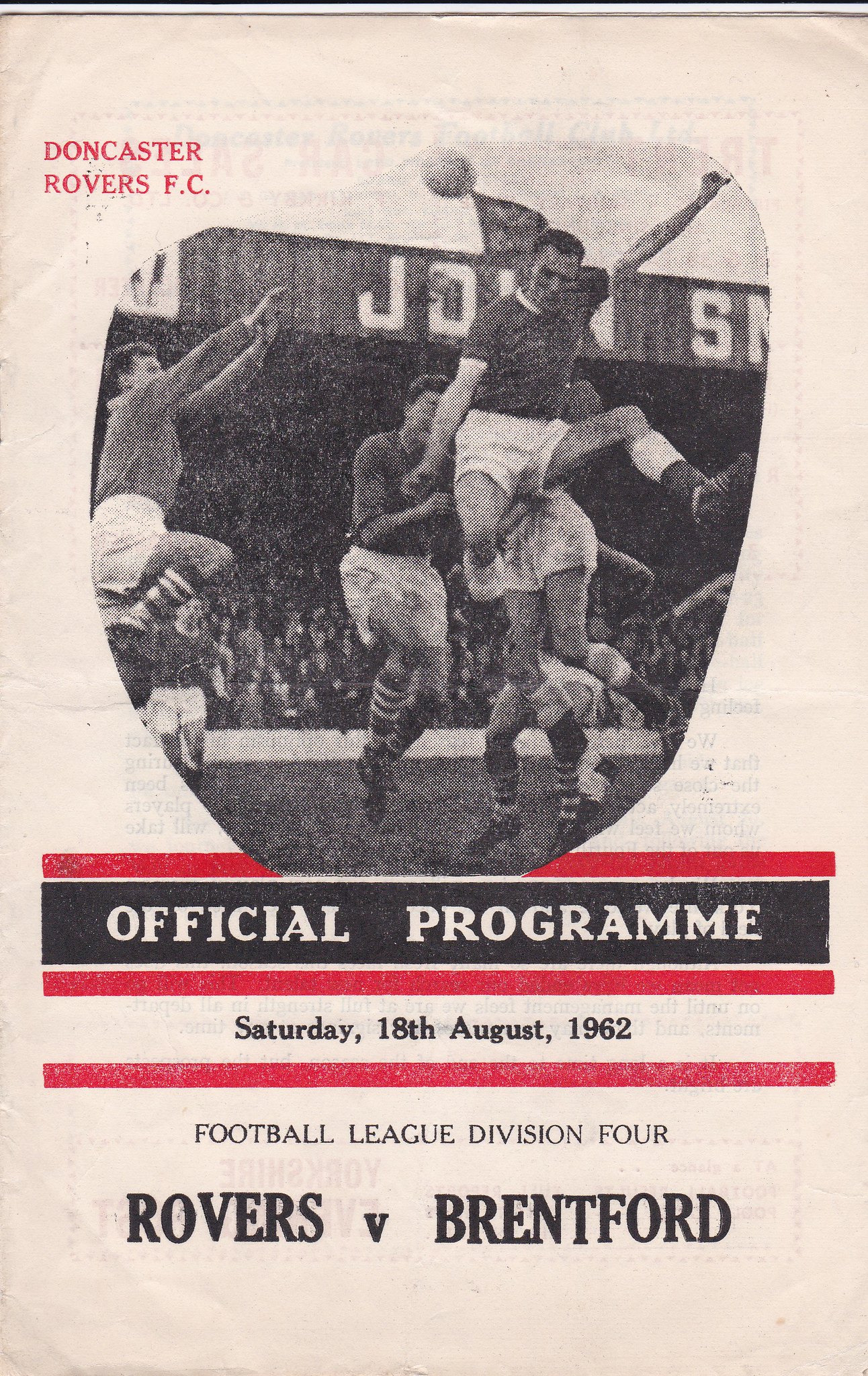This is a detailed description of a vintage soccer program for the Doncaster Rovers FC, dating back to August 18th, 1962. The entire program has an aged, browned appearance, suggesting it was once white. In the top left-hand corner, in small red letters, it reads "Doncaster Rovers FC." Just below this, there is a black-and-white photo featuring five players on a field, one of whom is jumping high into the air near a football. The scene suggests an energetic moment in a game, with the stadium and other players visible in the background. Below the photo, a red line separates it from a black banner that announces, in white letters, "Official Program." Further beneath, between two more red lines, the date "Saturday, August 18th, 1962" is displayed, along with "Football League Division IV" and the match-up "Rovers vs. Brentford" in black letters. The overall color of the program is a worn beige, tinted slightly pink, highlighting its vintage nature.